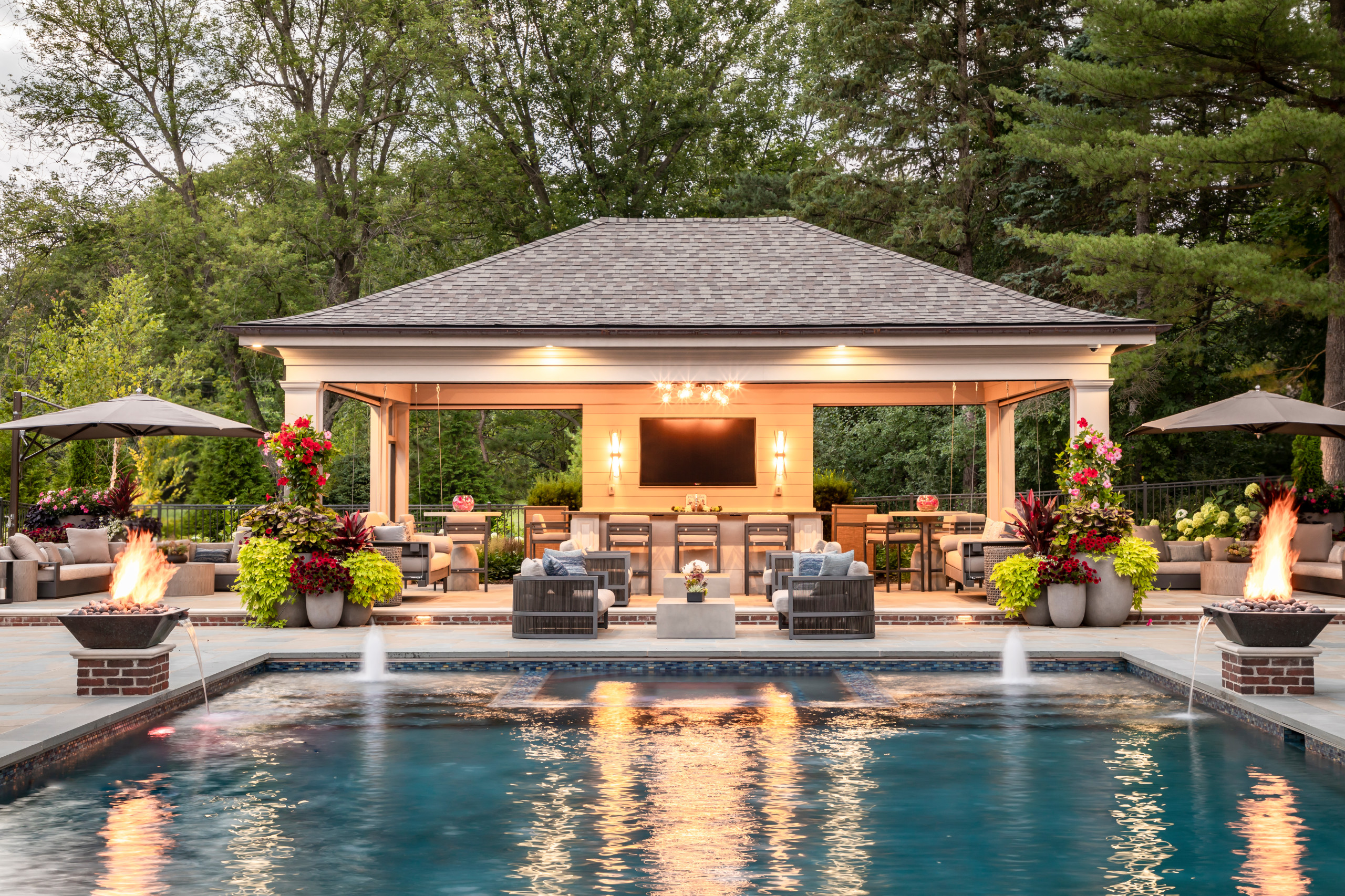The image depicts a lavish outdoor pool setting, most likely part of a high-end resort. The sizeable swimming pool is surrounded by elegant light and dark gray concrete tiles. Fountains and lit fire features on either side of the pool pour water gracefully into it. At the far end of the pool, there's a comfortable seating area with plush sofas adorned with numerous throw pillows, complemented by a gray end table. Beyond this, a pavilion with a light wooden roof houses a more social space, possibly including a bar and various tables and chairs. This area is illuminated, possibly by a chandelier, adding to the inviting ambiance. To the left, you see another cozy seating arrangement under an umbrella, accompanied by a fire pit that intriguingly incorporates a fountain element. On the left side, the fire pit, nestled on bricks, also spills water into the pool. The backdrop features a lush green landscape with trees and a black privacy fence for added seclusion. Additional chaise lounges and another umbrella area are visible to one side, along with a large patio area that includes various amenities such as a large screen TV, grills, and tall tables. The entire area exudes a sense of luxury and meticulous decoration, highlighted by vibrant flowers and multiple seating options under shaded sections.